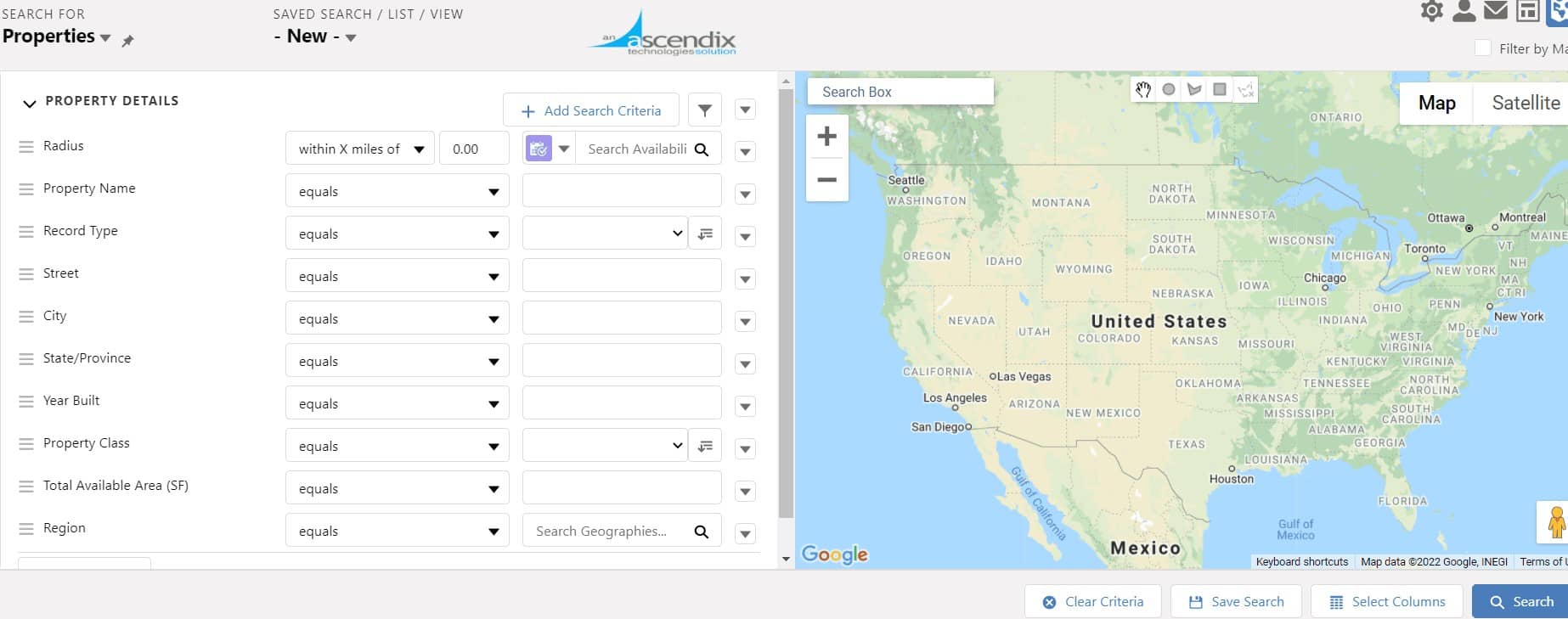This detailed caption describes a complex user interface for a real estate management platform, provided by Ascendix:

---

**Detailed Caption for Screen Interface Image:**

This image displays a screenshot of a dual-panel interface within a single cohesive digital experience, branded by the company Ascendix (spelled A-S-C-E-N-D-I-X). The top part of the screen prominently features the Ascendix logo alongside the company name.

On the left side of the interface is an input field section dedicated to property details. This area allows users to specify numerous parameters related to real estate properties, including:

- **Radius**
- **Property Name**
- **Record Type**
- **Street**
- **City**
- **State**
- **Province**
- **Year Built**
- **Property Class**
- **Total Available Space**
- **Region**

For each of these parameters, there is an associated filtering operator, currently set to "equals to" for all except 'radius.'

Adjacent to these fields on the right side are drop-down menus. These menus enable users to select appropriate values for each property attribute and operator, thus refining the search or data entry process.

The right side of the interface is dominated by a detailed map of the United States. This map showcases the names of all the states and highlights some of the major capital cities. Additionally, it clearly demarcates the international borders with Canada to the north and Mexico to the south, providing a comprehensive geographical context for users.